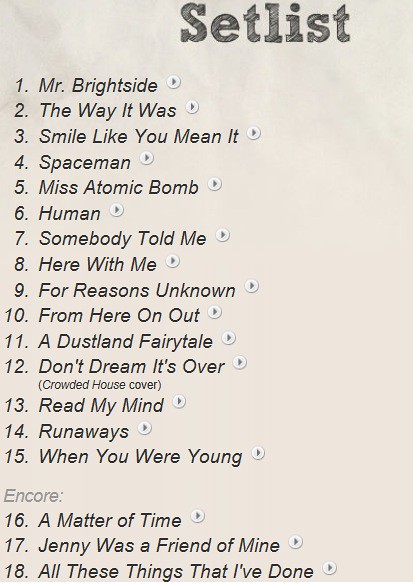This image depicts a neatly arranged set list against a light gray background. At the top center of the image, the title "Set List" is prominently displayed in large, bold, black letters. This bold header is followed by a list of 18 items, all written in black text. Each item on the list is preceded by its respective number and is accompanied by a small white circle containing a gray play arrow icon, suggesting the capability to play or select the item.

The list is as follows:
1. Mr. Brightside
2. The Way It Was
3. Smile Like You Mean It
4. Spaceman
5. Miss Atomic Bomb
6. Human
7. Somebody Told Me
8. Here with Me
9. For Reasons Unknown
10. From Here on Out
11. A Dustland Fairytale
12. Don't Dream It's Over (Crowded House cover)
13. Read My Mind
14. Runaways
15. When You Were Young

Beneath the initial 15 items, the word "Encore" is written in pale gray letters, signaling the encore section of the list. This section includes:

16. A Matter of Time
17. Jenny Was a Friend of Mine
18. All These Things That I’ve Done

The organization of the list, with its clear numbering and play icons, directs attention and provides an easy visual flow for the reader.